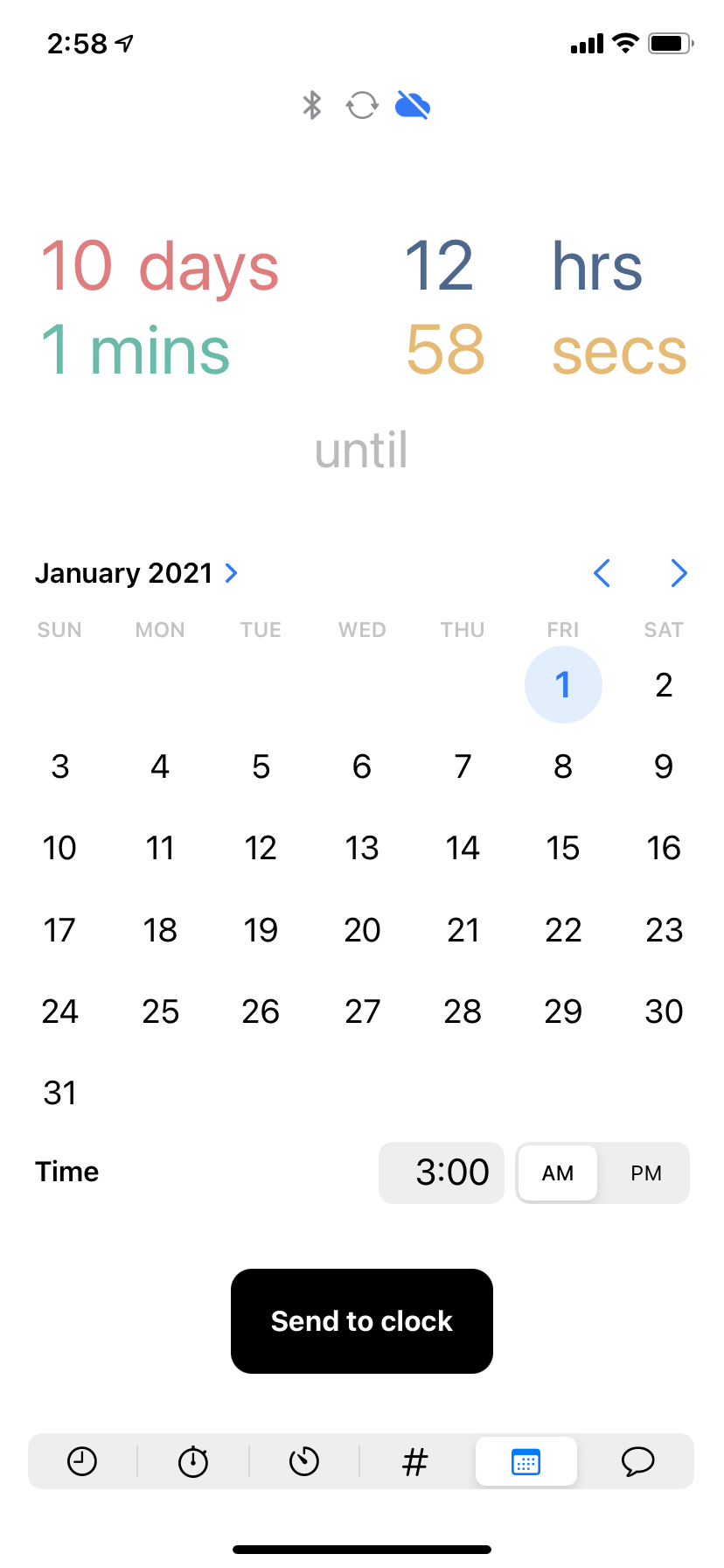Here is a cleaned-up and more descriptive caption for the image:

"Screenshot of a digital calendar display at 2:58 PM. The top left corner shows the current time, while the top right corner features icons indicating strong signal strength, cellular connectivity, and a nearly full battery. At the top center, there are additional icons: a Bluetooth symbol, a circular synchronization icon, and a blue cloud icon with a diagonal slash through it, indicating no internet connectivity.

Directly below these icons, a line displays '10 days' in red, '12 hours' in gray, followed by '1 minute' in green and '58 seconds' in orange, perhaps indicating time intervals. The calendar itself shows the month of January 2021, with the first day of January falling on a Friday and the last day, January 31st, occurring on a Sunday.

At the bottom of the calendar, the time is shown as 3:00 AM. Centrally located at the bottom is a prominent black button labeled 'Send to Clock.'"